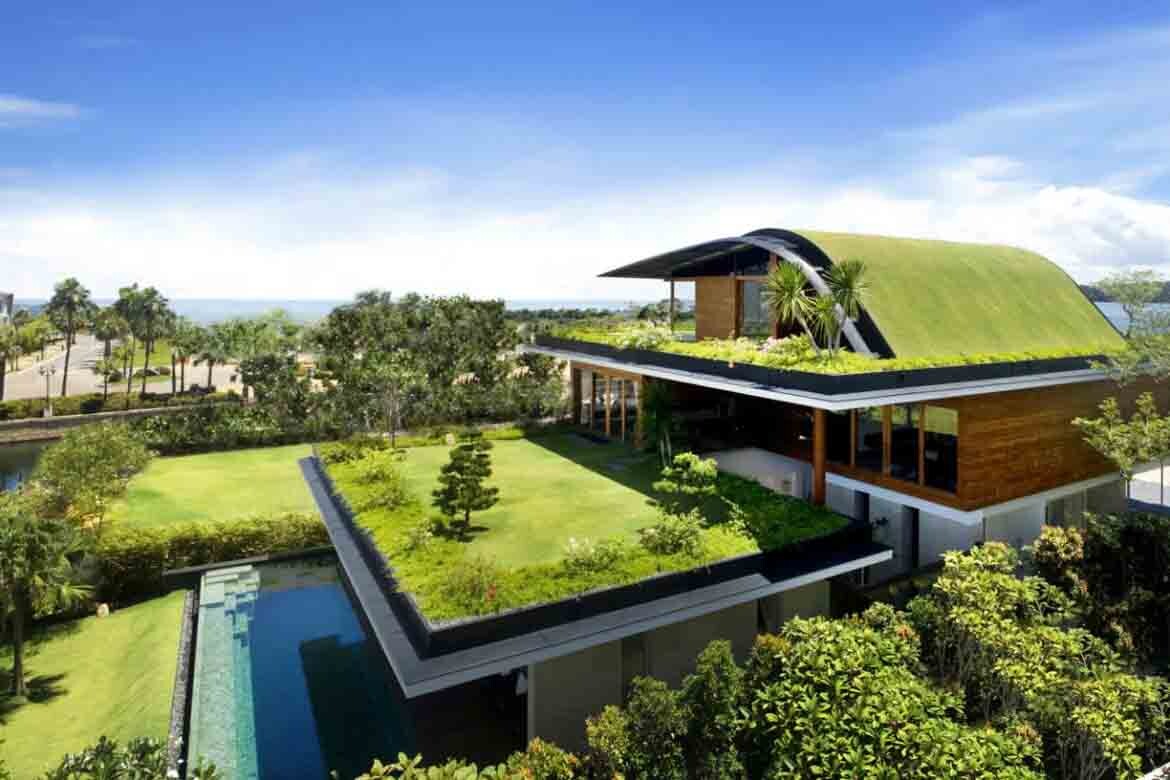In this aerial photograph, a strikingly modernistic, multi-story house is captured in the center, surrounded by lush greenery. This unique home boasts a green roof covered with neatly manicured grass and the second story features an expansive balcony adorned with palm trees and other foliage. The house itself is constructed with medium brown wood and accented with white, giving it a sophisticated yet natural aesthetic. 

The first floor of the house sits on a platform supporting a verdant lawn, which overlooks a crystal-clear blue swimming pool below. In the backdrop, a gray road lined with palm trees stretches towards the right side, leading the eye to a distant body of water surrounded by sand. The foreground is populated with various trees, contributing to the idyllic, verdant setting. The sky is a vibrant blue, filled with fluffy white clouds, adding to the picturesque quality of this unique, contemporary residence.